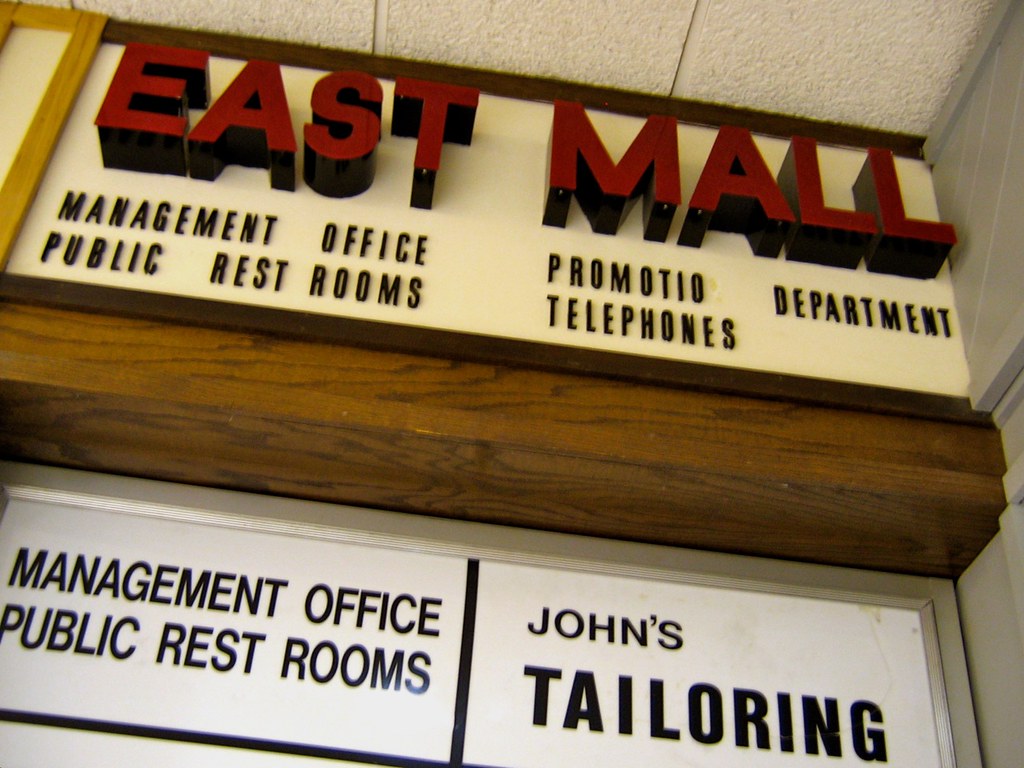A detailed caption for the image could be:

"In the interior of a mall, a directional sign hangs just below the white tiled drop-down ceiling. The sign, an off-white rectangular panel, features bold red text reading 'East Mall' at the top. Below in black text, it lists 'Management Office, Public Restrooms' on the left, and 'Promotion Department, Telephones' on the right. Underneath the sign, a darker brown wooden beam runs horizontally. Attached directly below this beam is another long rectangular sign. The left side of this second sign displays 'Management Office' with 'Public Restrooms' listed underneath. A dividing black line separates these from the right side, which prominently features 'John's Tailoring,' written with 'Tailoring' in thicker text."